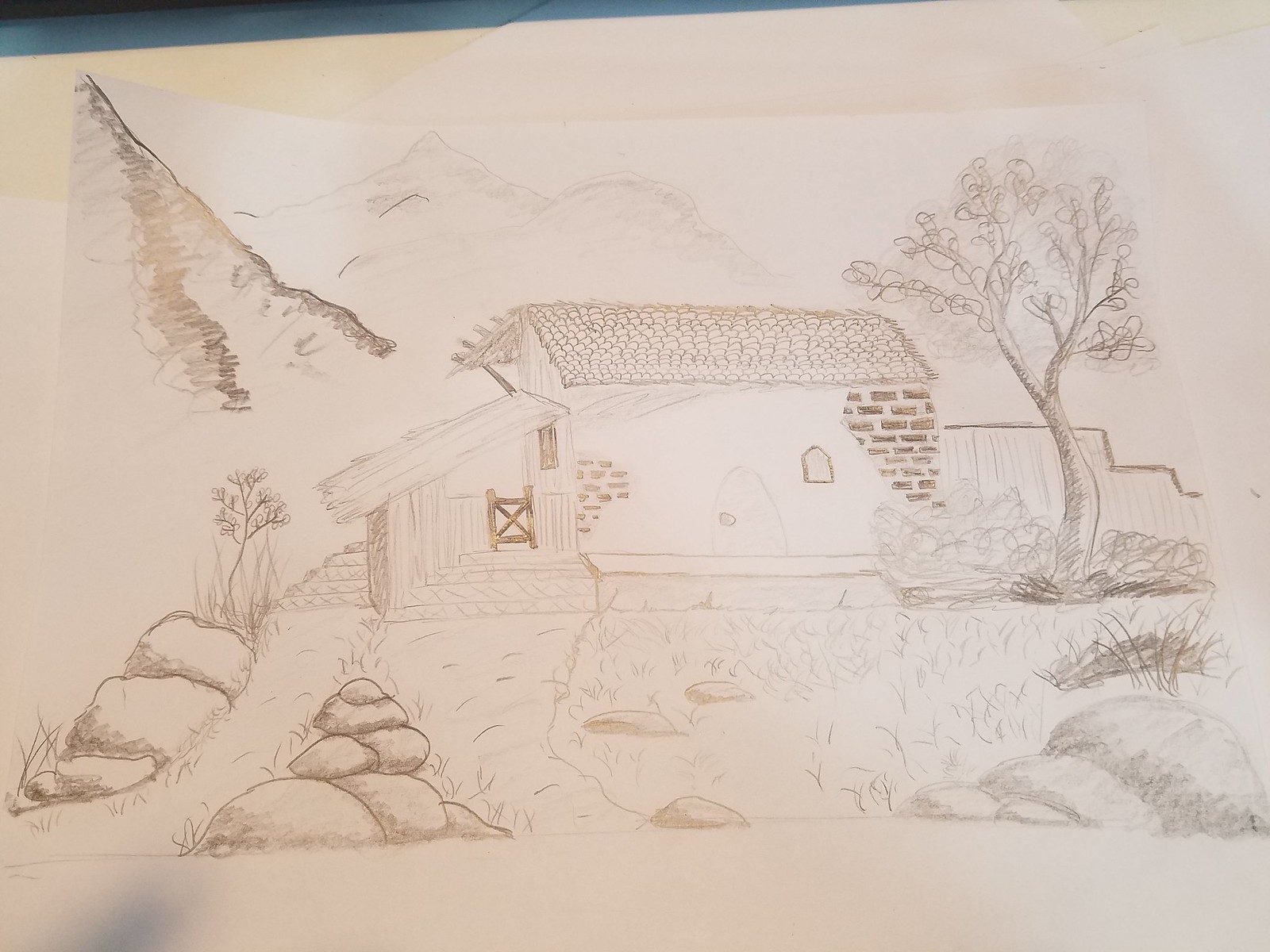This detailed drawing captures a rustic barn set in a picturesque landscape. The barn, with its brick exterior, boasts a roof textured with shingles, adding depth and realism to the structure. Attached to the left side of the barn is a lean-to with a sloped roof. To the right of the barn stands a leafy tree, providing natural contrast against the building. In the foreground, the yard features two distinct piles of rocks nestled among patches of grass. Further left, taller grasses can be seen, adding to the scene’s natural charm. The background is adorned with textured mountains, and birds soaring in the sky, adding an element of tranquility to the composition.